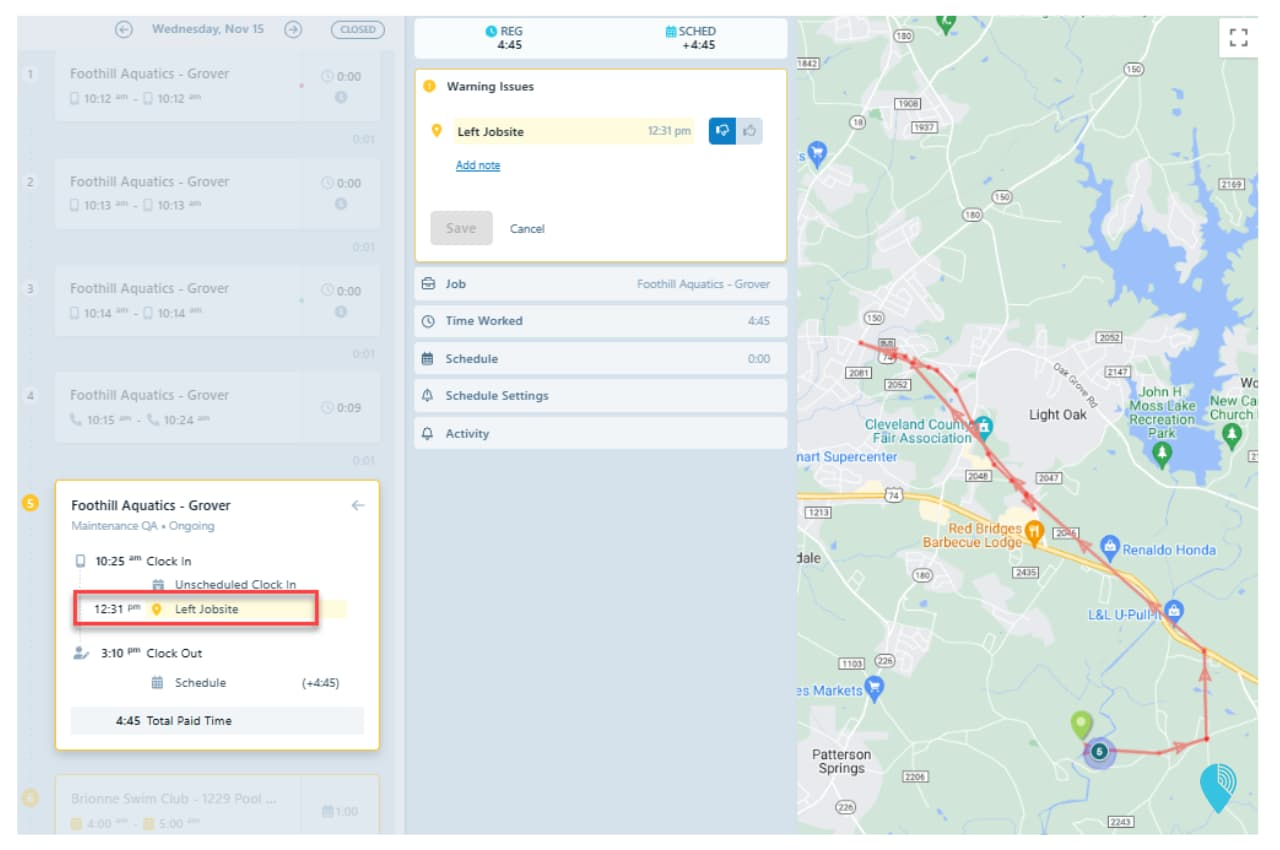The image is a detailed screenshot featuring what appears to be an interface reminiscent of Google Maps, although it is not explicitly confirmed. The map itself is positioned on the right side, occupying approximately one-third of the image, and is rendered in very light shades of green and blue. Various points of interest are highlighted on the map, including a notable mention of the "Cleveland County Fair Association" marked in blue font.

Central to the image is a prominent white square displaying a warning message that reads, "Warning: Issues left job site." Directly below this message, there is a categorization of items listed against a very light blue background, including "Job Time," "Worked Schedule," "Schedule Settings," and "Activities."

On the left side of the interface, a column is visible, and at the very bottom of this section, there is another white square. This square contains the text "Foothill Aquatics Grover," along with a schedule summary indicating entries such as "clock in," "left job site," and "clock out."